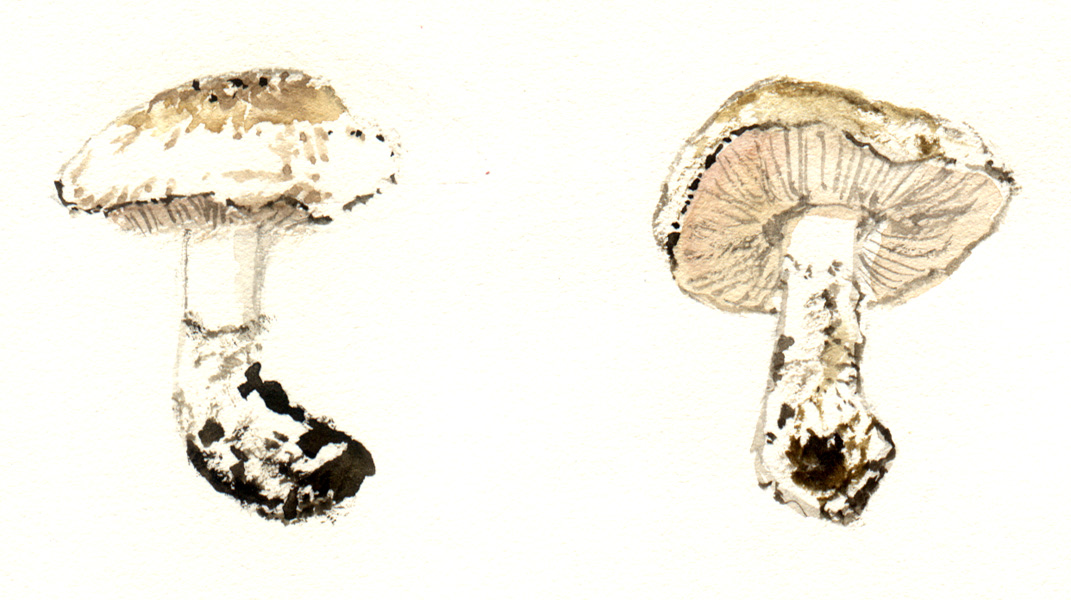This is a detailed hand-drawn illustration of two mushrooms on a solid white background, created with pencil and watercolors. The left mushroom is depicted from a side view, showcasing its irregularly rounded, speckled cap in shades of brown and beige, and a vertical stem that bends slightly to the right, covered in dirt at its base. The right mushroom, presented from a bottom angle, reveals the detailed, lined underside of its cap and a straighter stem, also displaying some brown speckles and dirt at the base. The artistic rendering features meticulous shading and texture to enhance the realistic appearance of the mushrooms, which appear slightly larger than life-size.